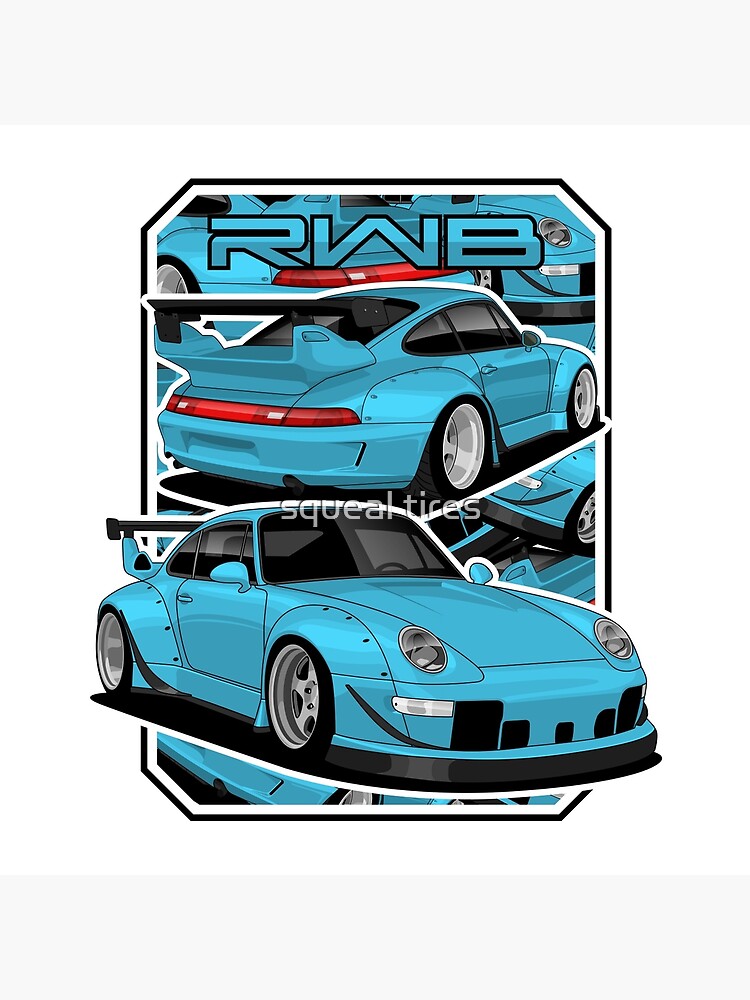The image is a detailed drawing of two sleek, Tiffany blue sports cars, resembling Porsches but without a distinct brand name. The upper car is depicted from the rear, showcasing a red line of taillights, side mirrors, a tinted windshield, a prominent spoiler, and the letters "RWB" in thick, comic book-style font colored in the same blue with a black outline above it. The lower car is oriented towards the right lower corner and is viewed from the front, highlighting the headlights and the clean, aerodynamic design, all in a deep, electric blue hue. The image has rounded corners and features a black outer edge with a white inner border, creating a framed effect. There is also a watermark across the middle that reads "Squeal Tires," hinting at it being an advertising image.